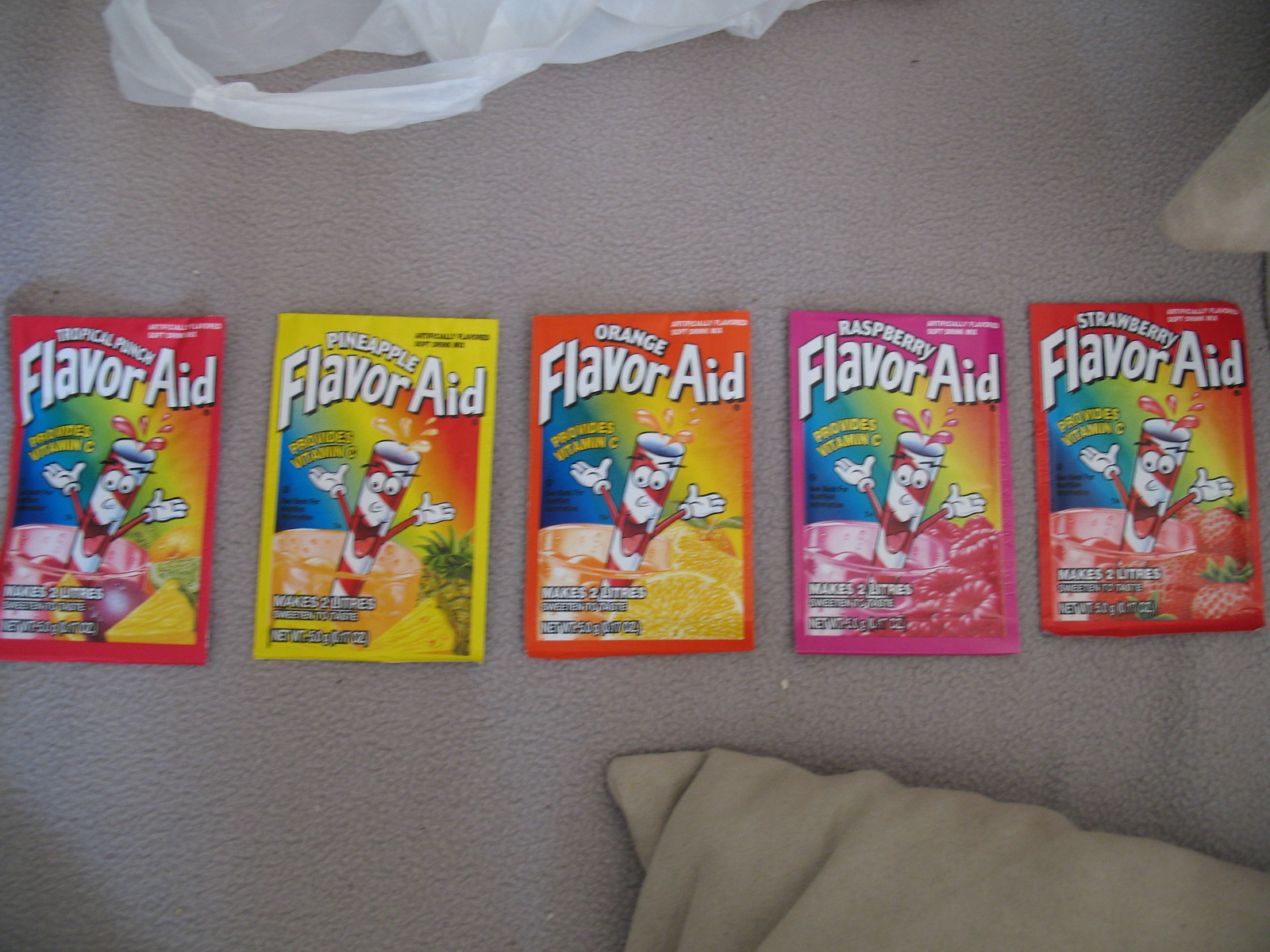This image features five Flavor-Aid drink mix packages, each distinctively colored to correspond with its flavor, neatly laid out on a light gray background that appears to be part of a Sherpa quilt. In the upper left corner, there is a plastic grocery sack handle visible, and a beige pillow is partially seen in the bottom right corner. From left to right, the packages are:

1. **Tropical Punch**: This package has a red outer border. It showcases a glass character with a striped red and white straw, featuring eyes, white-gloved hands, and drops coming from the top. It also indicates that it "provides vitamin C" in yellow text and has vivid fruit imagery below the character.
   
2. **Pineapple**: The second package is yellow and follows a similar design, with the glass character now in an orange glass, holding an image of pineapple.

3. **Orange**: The third package is orange with the glass character depicted in a darker orange juice glass, suitable for its flavor.

4. **Raspberry**: The fourth package is pink, featuring the glass character in a raspberry-colored glass representing the raspberry flavor.

5. **Strawberry**: The final package is bright red, with the glass character appearing in a light red juice glass, embodying the strawberry flavor.

Each packet states it "provides vitamin C," can make two liters of beverage, and includes fruit imagery related to its flavor.